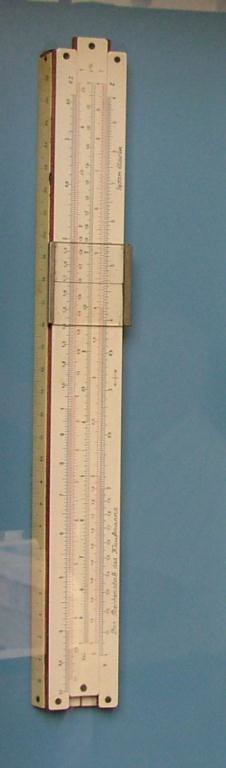This photo captures a device that closely resembles a multi-functional ruler, set against a light blue background. The background fades away into a lighter hue towards the upper right corner, suggesting it may be a piece of paper serving as a backdrop. The ruler-like device is predominantly rectangular, but it features additional rectangular elements that jut out from the top, though they do not extend along its entire length. 

The bottom of the device has a cut-out section, possibly indicating it slides up and down. A transparent material, possibly plexiglass, covers a section in the middle, enhancing its multi-functional aspect. On the left side of the device, another ruler appears to overlap partially, adding to the complexity.

In the lower left corner, there is a noticeable glare, which could be due to a photographic artifact or an actual piece of paper affixed to the device. Towards the bottom portion of the rectangle, there are three punched holes, while another hole is located on the left side, suggesting it might be designed for hanging or securing the device.

Throughout the device, there are numerical markings, typical of rulers, but the exact details are difficult to discern from the photograph.